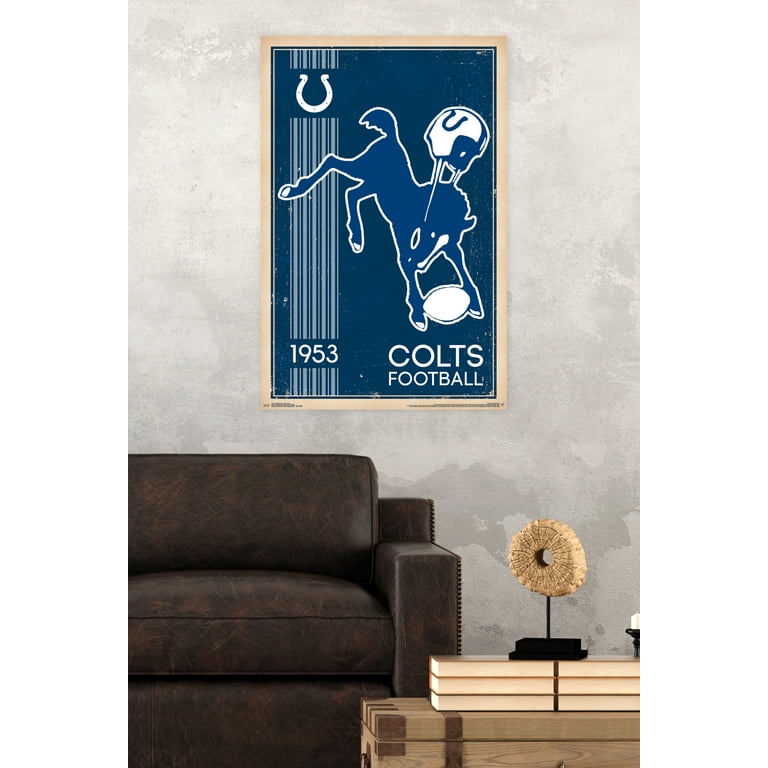This is a vertically oriented, realistic photograph of a living room area. In the bottom left corner, there is a brown leather couch, of which only its right side is visible. In front of the couch stands a light wood chest functioning as a coffee table, adorned with about six books stacked on top. Atop the books is a small black stand holding a wicker circle sculpture, resembling a lollipop made out of twine. To the right of these items, there is a black candle stand with a short white candle.

The background features a textured grey wall. Centrally mounted on this wall is a striking blue poster bordered in tan, measuring approximately a foot and a half in width by two to three feet in height. The poster prominently displays the date "1953" in white at the bottom left and the text "Colts Football" in white at the bottom right. An upside-down white horseshoe, symbolizing the Colts logo, appears at the top left. The poster also showcases blue stripes along the left side and features an illustration of a bucking colt. The colt is depicted in blue with a white outline, wearing a white football helmet marked with a blue 'U' and clutching a white football between its front legs.